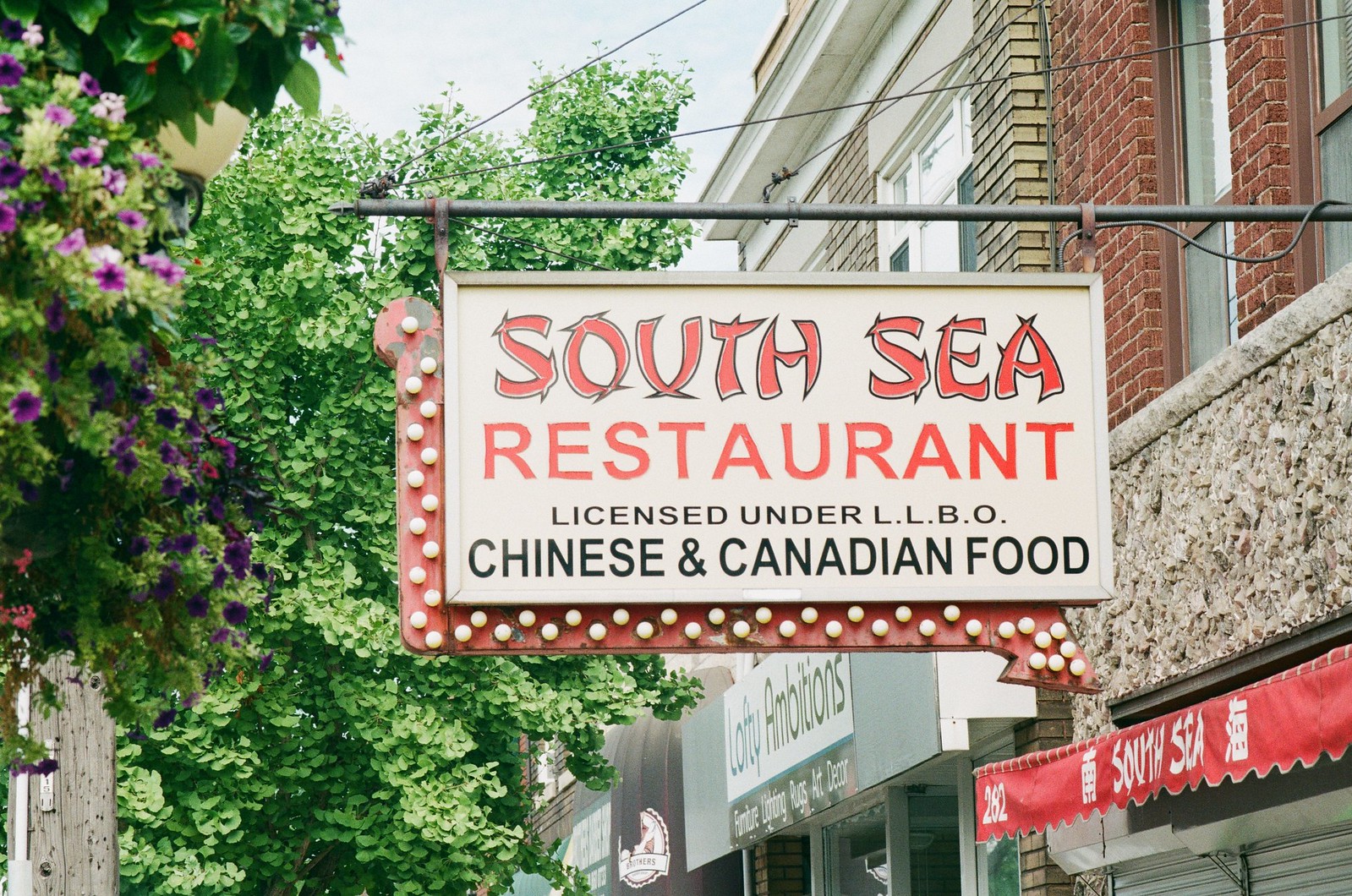This horizontally aligned, landscape-oriented color photograph captures a detailed view from the sidewalk, looking up at an outdoor sign hanging above a restaurant. The sign, projecting from a dark metal pole affixed to the side of a stone and red-bricked commercial building, reads "South Sea" at the top in red text outlined in black, followed by "Restaurant" in red, and "Licensed under LLBO, Chinese and Canadian Food" in black underneath. A red arrow bordered with small white lights points to the bottom right, presumably indicating the restaurant’s entrance. Below this sign, the building features a red and white canopy with "South Sea" printed on it. The left side of the image shows lush green trees with purple flowers against a partly sunny sky adorned with blue and white clouds, intersected by telephone wires. The setting conveys a quaint urban scene during the day with additional nearby shops implied in the background.